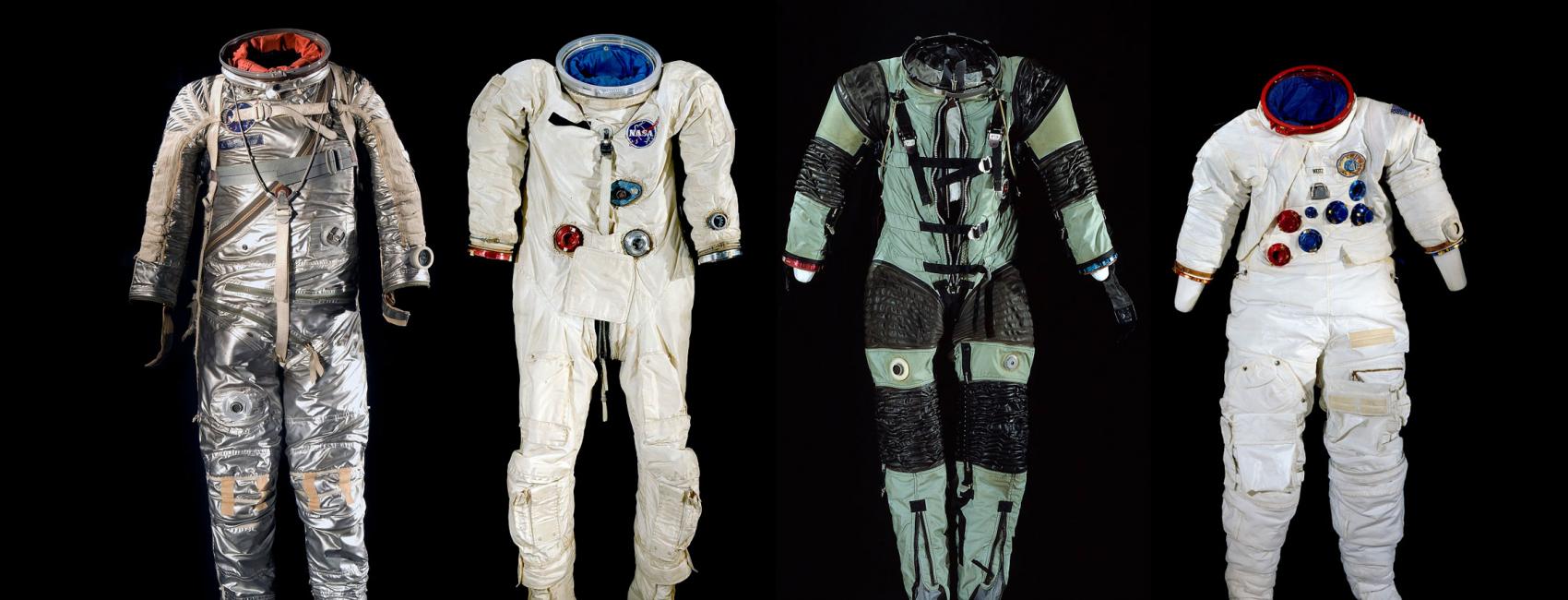The photograph features four distinct spacesuits, displayed against a black background. The first suit on the left is highly reflective with a silver, almost foil-like finish, and appears aged. It has brown straps and a silver ring at the neck for helmet attachment, revealing red material inside. The second suit, to its right, is a white suit featuring a NASA logo on its left chest. It has several ports on the front in red, white, and blue for attaching hoses. This suit also has blue material inside and rings around the cuffs, one red and one silver. The third suit is primarily teal green with black stripes across the arms and legs, giving it a segmented appearance. It also has a neck ring but the internal cloth is not clearly visible. The fourth and final suit is another white suit, sturdier-looking with a red anodized metal neck ring. It has multiple ports of different sizes on the chest, likely for various life support connections, and blue material inside.